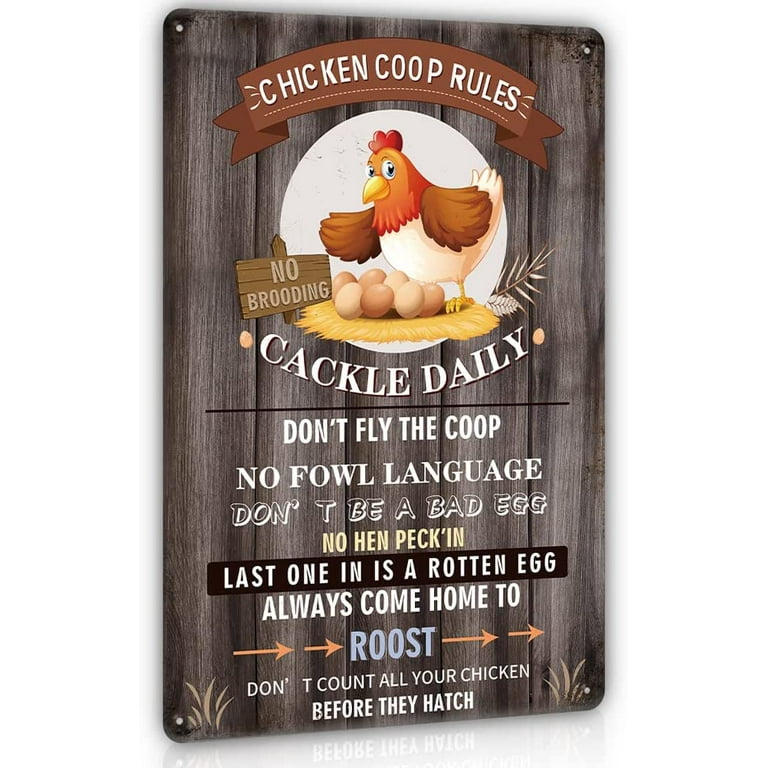The image is a digital rendering of a wooden plaque with a light gray background, designed to look like it has a wood texture and four rivets, one in each corner. At the top, the plaque boldly states "Chicken Coop Rules." Below this title, a cartoon chicken is depicted perched above seven eggs, surrounded by some straw. The sign humorously lists a set of whimsical rules: "No Brooding," "Cackle Daily," "Don't Fly the Coop," "No Foul Language" (with a pun on "foul"), "Don't Be a Bad Egg," "No Hen Pecking," "Last One in Is a Rotten Egg," "Always Come Home to Roost," and "Don't Count All Your Chicken Before They Hatch." These playful, chicken-themed phrases offer words of wisdom and are perfect for kitchen decor.